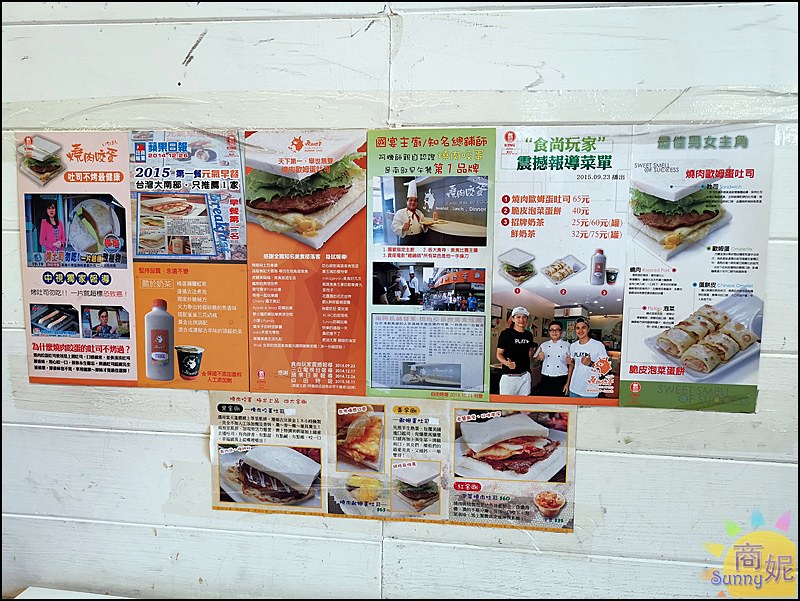In this color photograph, a dirty, off-white tiled wall is covered with six large posters aligned in a row at the top, each varying in color from orange, peach, and red to white and green. Below them hangs a smaller, folded poster. The posters predominantly feature images of food items like sandwiches and rolls, as well as beverages, and include pictures of men in chef or cook uniforms, suggesting they could be advertisements for a restaurant or food products. All the text on the posters is written in small print using Chinese characters.